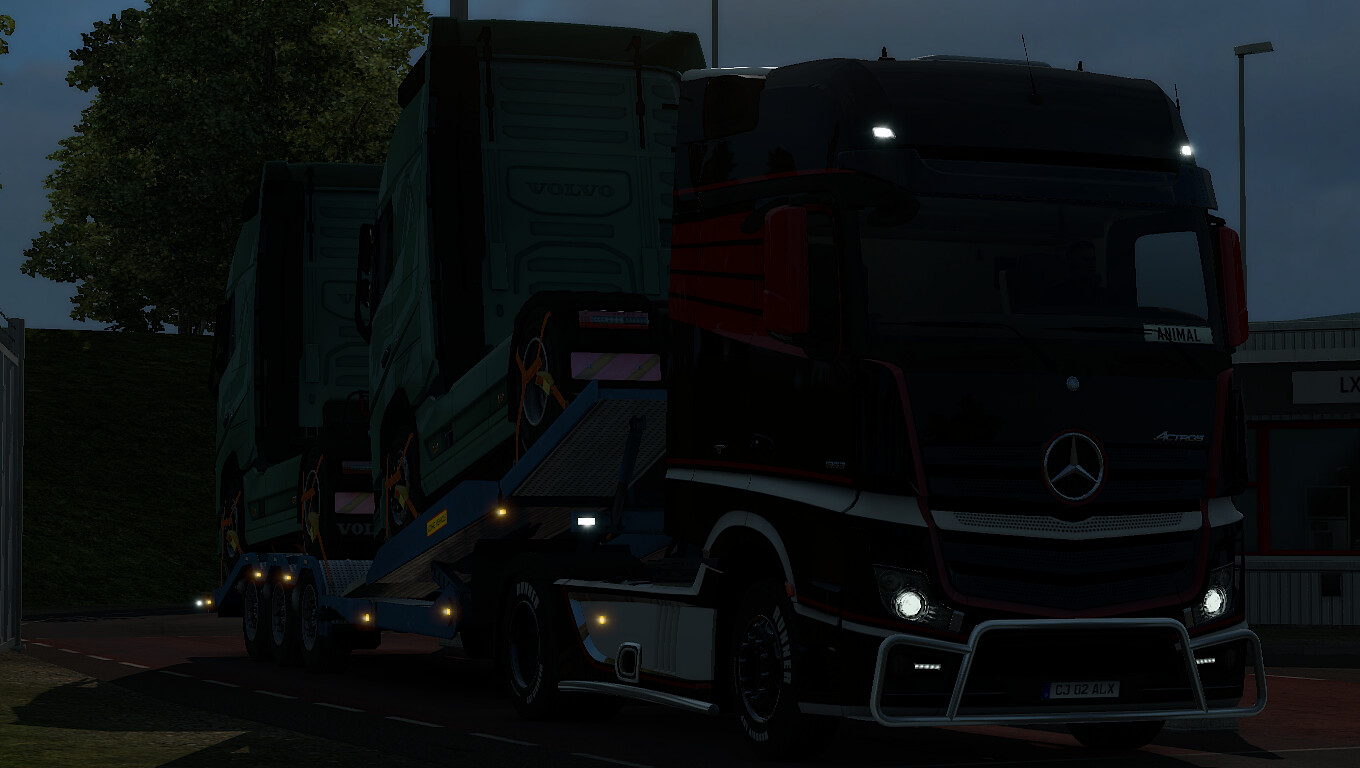In this computer-generated, nighttime image, we see a parked, European-style short-nosed Mercedes semi-truck with a compact cab. The semi-truck, painted black with a red stripe and featuring a prominent chrome Mercedes emblem in the center of the cab, stands out despite the very dark setting. The truck’s headlights, positioned both on the bottom and above the cab, illuminate parts of the scene. Behind it, the semi-truck is hauling two more Mercedes semi-trucks, which are aqua blue in color. These trucks are loaded back-to-back on a trailer, emphasizing their minimalist cab design without any cargo attached. A tree is visible in the left-hand side of the image against a backdrop that hints at an evening sky, adding to the moody atmosphere.